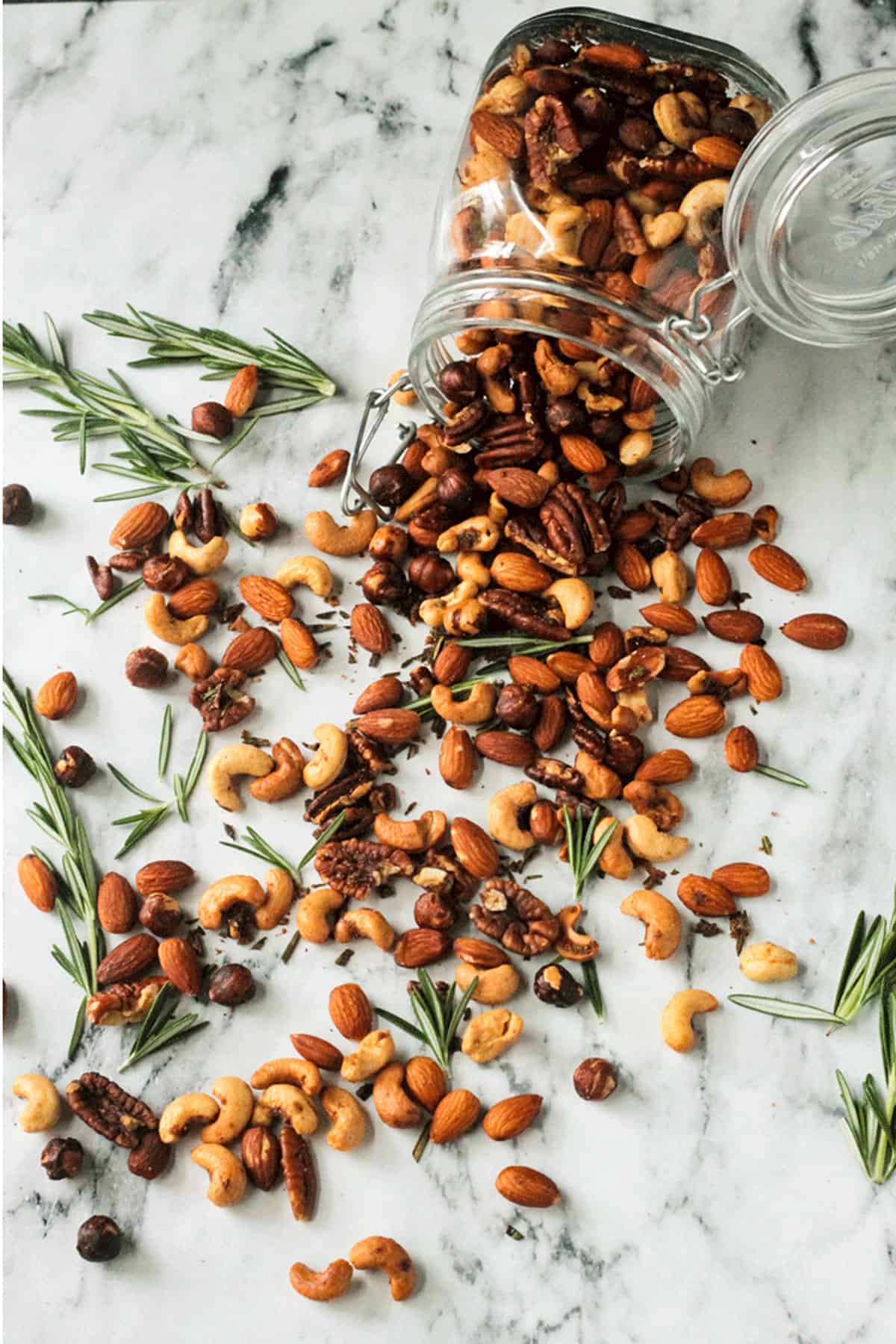This close-up photograph features a glass mason jar with a metal hinge, lying tilted on its side on a black and white marble-patterned countertop. The jar is positioned towards the upper right corner, spilling out an assortment of mixed nuts, which include pecans, almonds, cashews, and peanuts, along with some dark-colored round nuts. The scattered nuts appear dense near the jar and gradually sparse as they spread towards the middle and lower left corner of the image. Adding a decorative flair, small green leaves or herbs are interspersed among the nuts, providing a pop of color against the monochromatic backdrop. Although the jar lid has an inscription, it is not legible in the photograph, and no other identifying text is present.